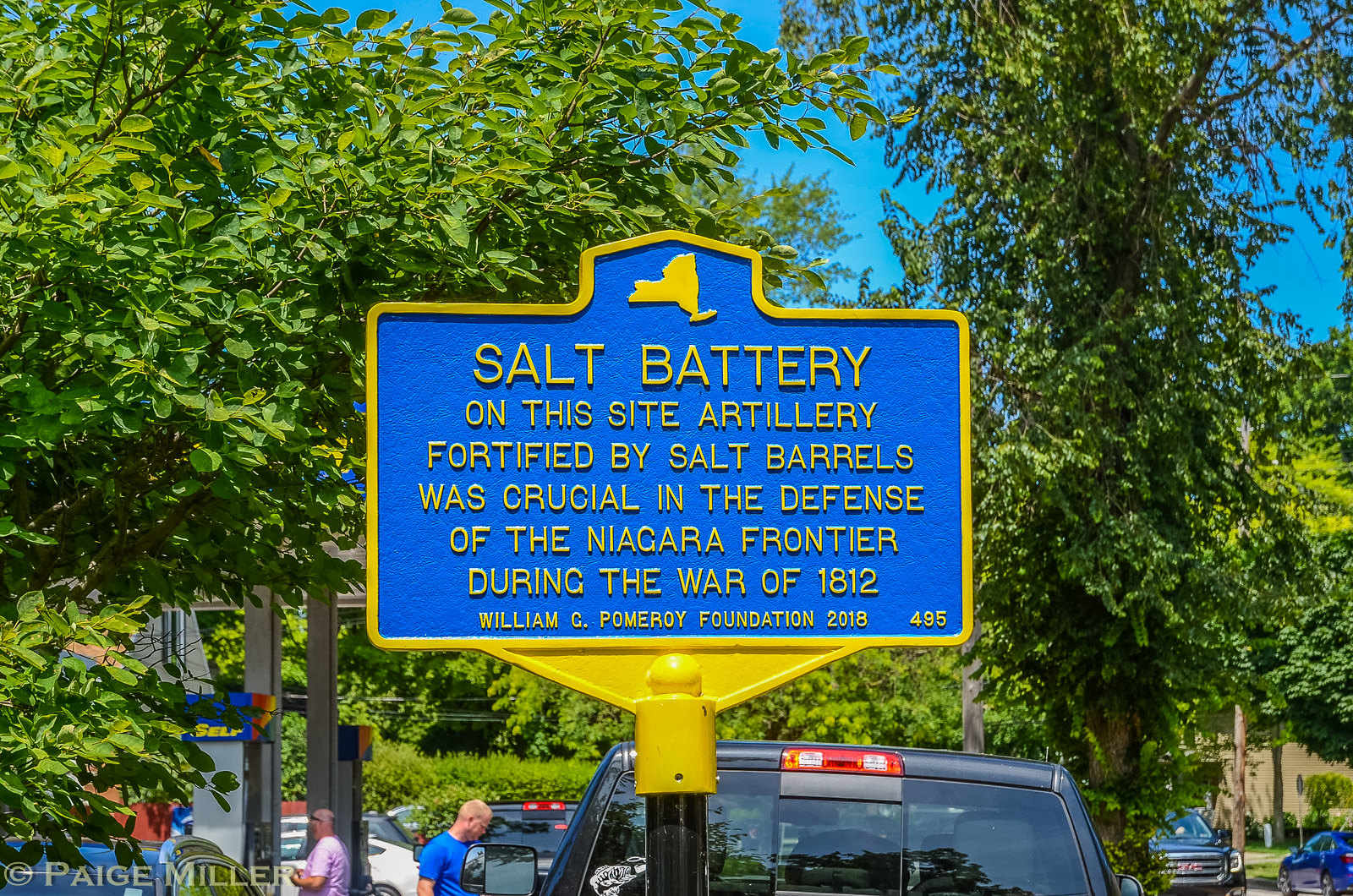This detailed outdoor image, set in a lush New York state park, features a prominent blue metal sign with a yellow border and a small depiction of the state of New York at the top. The text on the sign, written in yellow, reads, "Salt Battery. On this site, artillery fortified by salt barrels was crucial in the defense of the Niagara Frontier during the War of 1812. William C. Pomeroy Foundation, 2018," and is followed by the number "495" at the bottom right. The sign is mounted on a metal post and framed against a backdrop of trees with vibrant green leaves. In the foreground, a black truck with a red light on top is parked along with several other vehicles visible toward the bottom and right of the frame. People are seen to the left of the truck. Additionally, there is a subtle mention of the copyright symbol and the name Paige Miller at the bottom left corner of the photo.